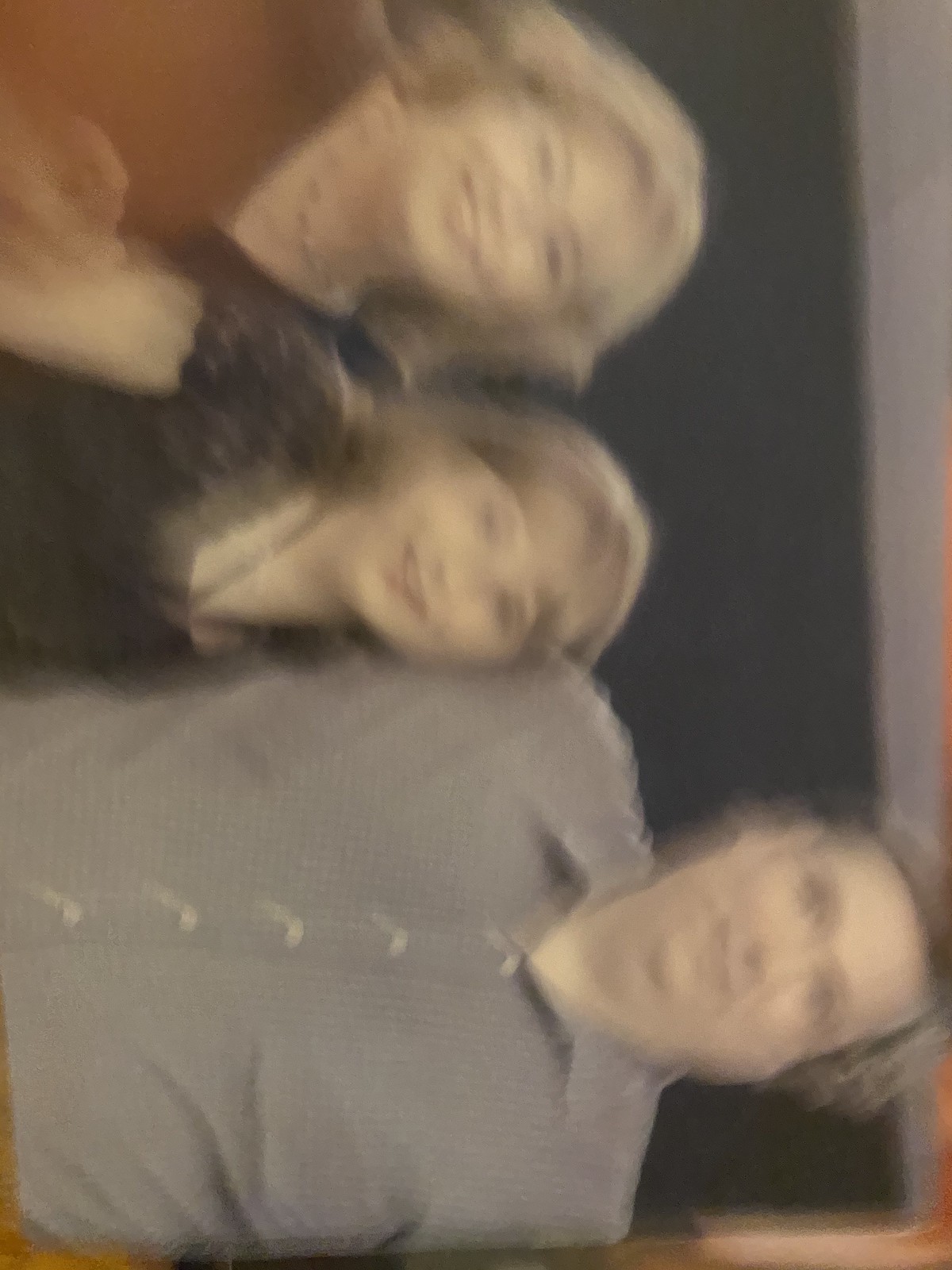This is a sideways, very blurry image featuring a group of three individuals—a man and two women. The man, who is quite large with slightly long, graying hair, is wearing a gray button-down shirt and is looking directly into the camera with a neutral expression. He has his arm around one of the women while gently placing his hand on the other woman's head, possibly as a sign of affection. One of the women, who is wearing black and has a slight smile, is positioned next to him. The other woman, dressed in red and displaying a much broader smile, is the recipient of the man's affectionate hand on her head. Despite the blur, these subtle interactions hint at a close, possibly familial or friendly relationship among the trio.